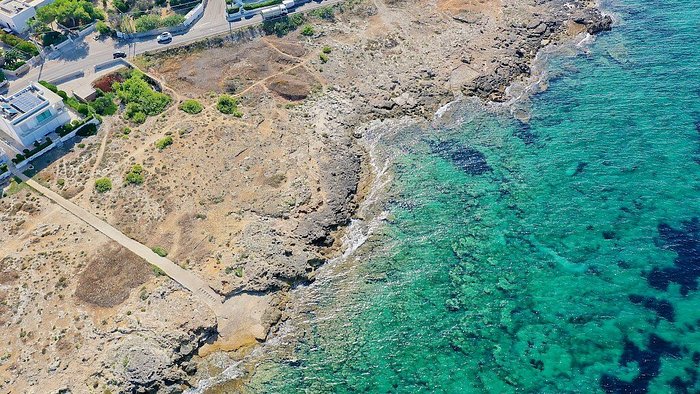This aerial photograph captures a striking landscape combining both land and sea. On the right side, the image showcases an expanse of clear blue and greenish water, so transparent that coral formations are visible beneath the surface. Adjacent to the water, dark green rocks form a rugged shoreline. Transitioning to the left, the coastline gives way to brown, arid land punctuated by a dusty road that meanders through the area. Vegetation, including patches of green plants and trees, is sprinkled amidst this barren terrain. More inland, houses—including a notable large white structure that appears to be a two-story home—are visible alongside the road. This pathway connects the beach to the inland, indicating human habitation and activity in the scene. The blend of natural features and human elements under the daylight creates a vivid and detailed representation of this tropical locale.